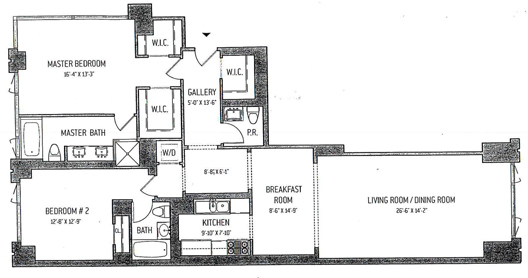In this detailed architectural floor plan of a residence, the layout reveals thoughtfully designed spaces delineated by precise lines and accented with black type for clarity. The residence features a living room and dining area, gracefully separated by folding doors that open to the outdoors, creating a seamless indoor-outdoor connection. Adjacent to the dining area is a cozy breakfast room that provides a peaceful spot for morning meals.

From the breakfast room, a small hallway leads into a gallery, which serves as a transitional space bridging various parts of the home. This gallery extends towards the front entrance, where visitors are greeted by a walk-in closet and a convenient powder room. The master suite, accessed by turning right upon entering the front door, boasts a luxurious master bedroom. This room offers ample storage with two walk-in closets—a smaller one for immediate needs and a larger one for additional storage. The master bathroom complements the suite with a bathtub, a shower, and dual sinks, ensuring maximum comfort and functionality.

Continuing along the gallery from the front entrance, another small hallway to the right houses a practical washer and dryer setup. Beyond this utility area, there is a secondary bathroom featuring a bathtub and a single sink, alongside a well-appointed bedroom equipped with a sliding door closet, ideal for a child or guest.

The breakfast room also offers access to a galley kitchen, outfitted with essential appliances, including a range and a sink. This kitchen is designed exclusively for access from the breakfast area, enhancing the intimate and efficient layout of the home. Overall, the floor plan presents a harmonious blend of private and communal spaces, expertly crafted for comfort and practical living.